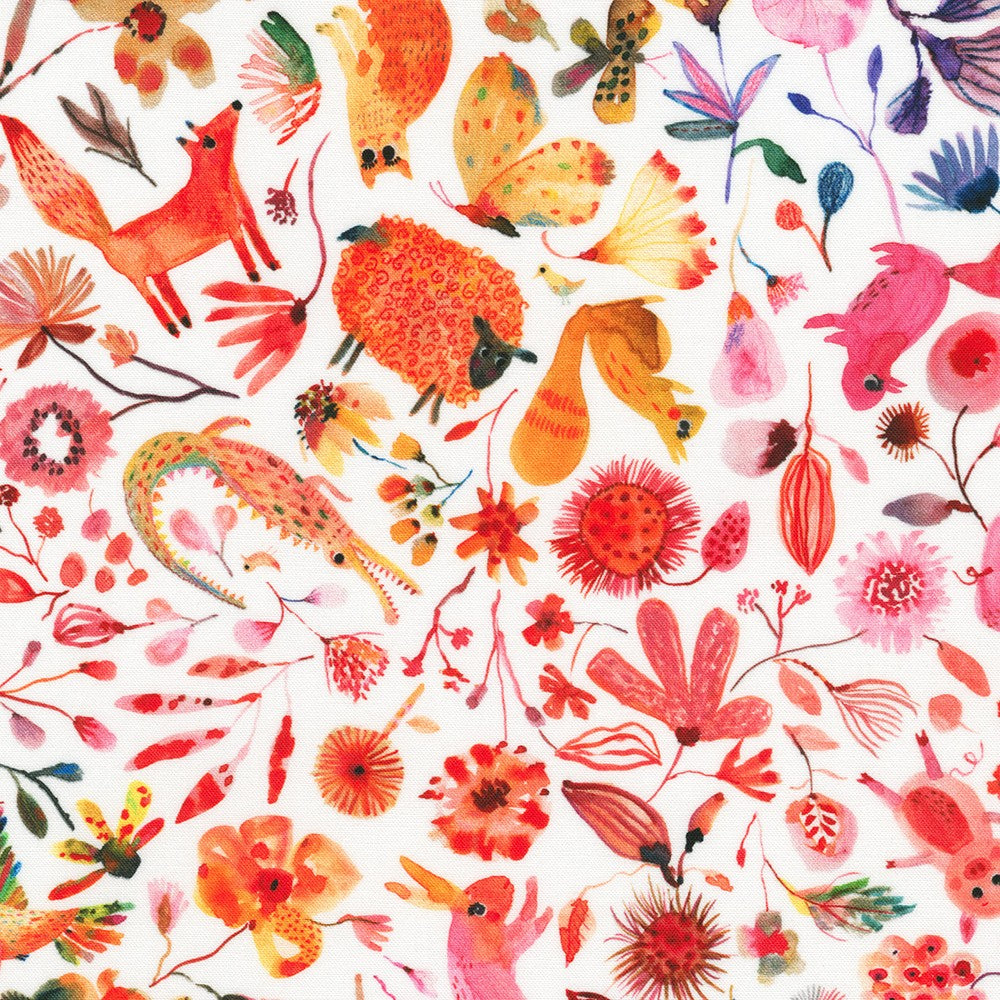This vibrant, color photograph depicts a whimsical, vintage-inspired pattern that could be seen on wallpaper, fabric, or a tablecloth. The pattern showcases an array of illustrated animals and blooming flowers, all playfully arranged in a spectrum of colors transitioning from pinks and reds on the left, through oranges, yellows, and back to pink, and then purples. Set against a white background, the scene includes cartoonish creatures like a fox with its tail up, an orange-colored alligator on its side, and a pink rabbit emerging from the bottom. There's also an upside-down cat, squirrel, and pig, as well as another pink squirrel at the top right. Butterflies with beige wings outlined in red and a variety of flowers from thistles to blooms in shades of red, orange, pink, blue, and purple fill the spaces, along with scattered green leaves. The random orientation of the design elements means it can be viewed from any angle, adding to its playful charm.